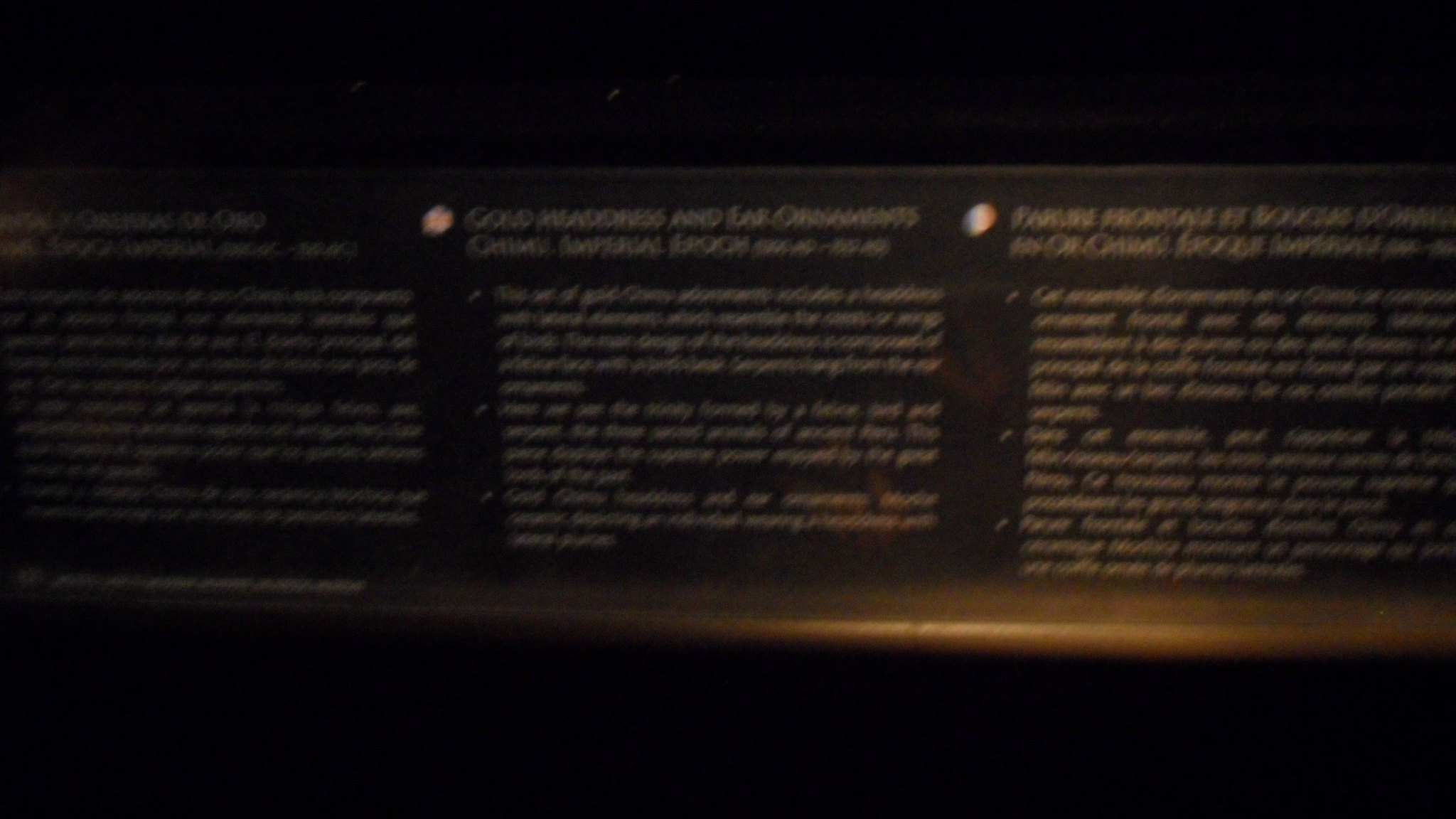This image depicts the back panel of an unidentified electronic device or cable box. The focal point is a black label with white text, though the poor image quality renders the specific details largely unreadable. The label appears to contain information in three different languages, with the phrase "GOLD MADRAS" (or possibly "GOLD HEADDRESS") somewhat discernible in the center section. The photograph is notably blurry and grainy, with heavy smudging on the label. The background and edges of the photo are predominantly black, and a light source from the right side reflects faintly across the bottom, adding to the overall obscurity.